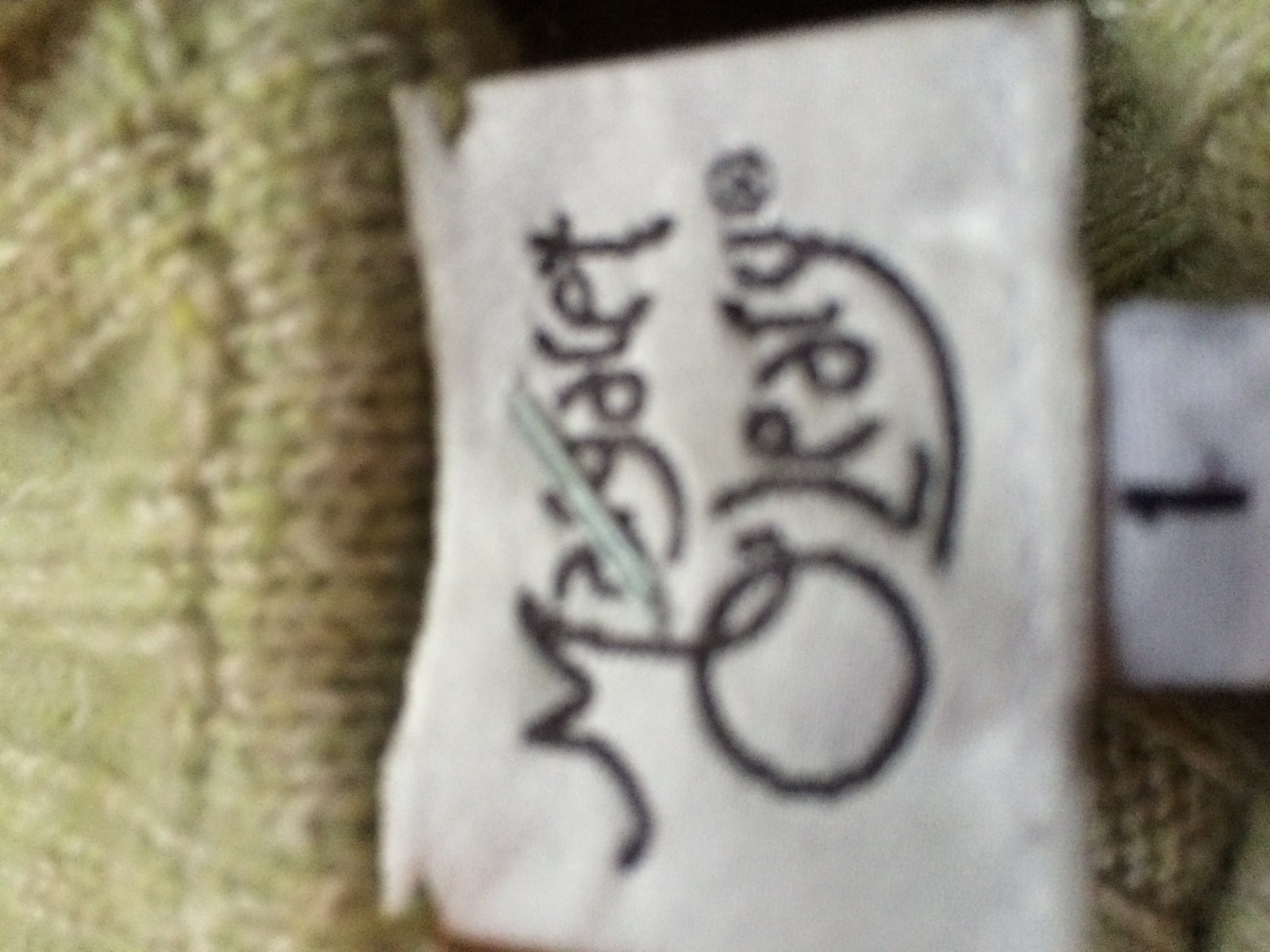The image displays a very blurry close-up view of a tag on a garment, positioned sideways. The tag, which is white and features cursive black text, reads "Margaret O'Leary," with a trademark symbol following the name. "Margaret" seems partially obscured by a clear tube or object. The tag is attached to a coarse, multi-colored sweater primarily composed of shades of beige, olive green, pink, and white. The sweater appears to be cable-knit, showcasing various knitted textures. Beneath this prominent tag is another smaller white tag indicating the size, marked with the number "1" in black text. This entire fabric item seems to be situated on a tan-colored or light gray blanket, contributing to the blurred appearance of the overall scene.